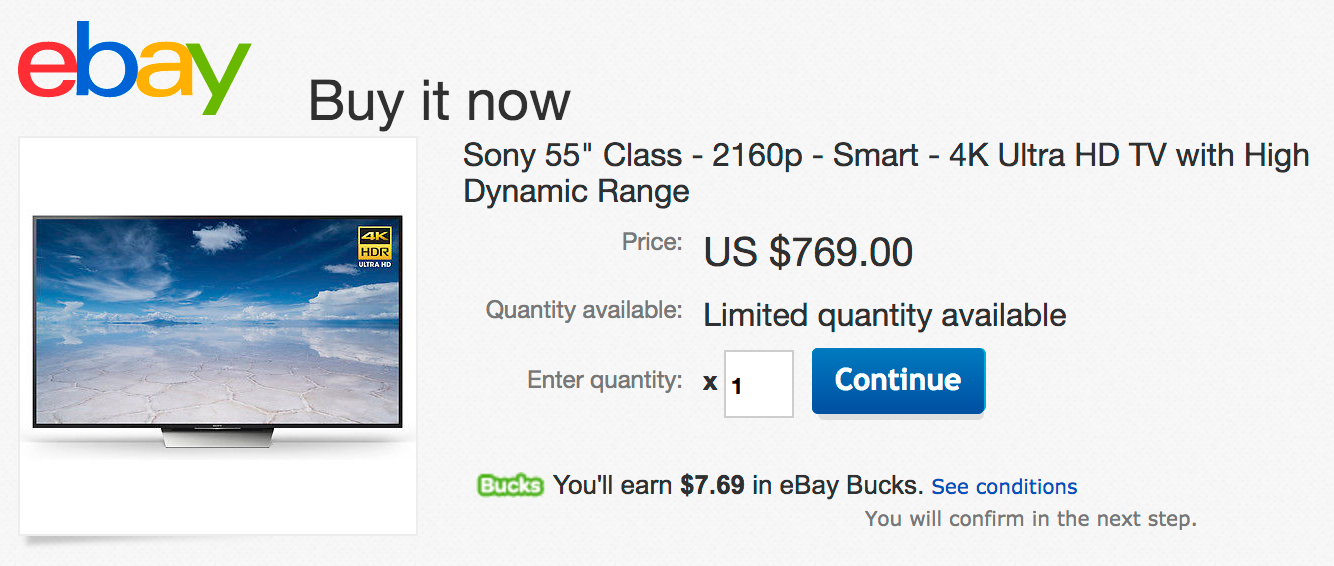This is a detailed screenshot from eBay's website. The display is rectangular, approximately twice as wide as it is tall, set against a light bluish background. In the top left corner, the iconic eBay logo is displayed with large letters: a red 'e', blue 'b', yellow 'a', and green 'y'. Just below and slightly to the right is the bolded black text "Buy It Now."

Further down, the product description is detailed in black text which reads: "Sony 55-Inch Class - 2160p - Smart - 4K Ultra HD TV with High", continuing on the next line to the left with "Dynamic Range." Directly below "Range" in smaller black text is the word "Price", followed by a prominent "US $769."

To the left, small text indicates "Quantity available," with a bold statement "Limited quantity available" underneath. Further left again, in small black letters, it says "Enter quantity," next to a small black 'x' and a bordered white square containing the number '1'. Adjacent to this is a blue tab with the word "Continue" in white.

Moving down to the left side of the screen is a green-bordered area with the text "Bucks" in white lettering. Below it in black, it reads "You'll earn $7.69 in eBay Bucks," followed by a blue link that says "See conditions." Below this section, another black text states, "You will confirm in the next step."

On the left side, beneath the eBay logo, is an image of the TV inside a bordered area. The TV picture has a gold sticker on the top left corner with "4K HDR." The screen display features a scenic image with the bottom half depicting a desert and the top showing a sky with some clouds.